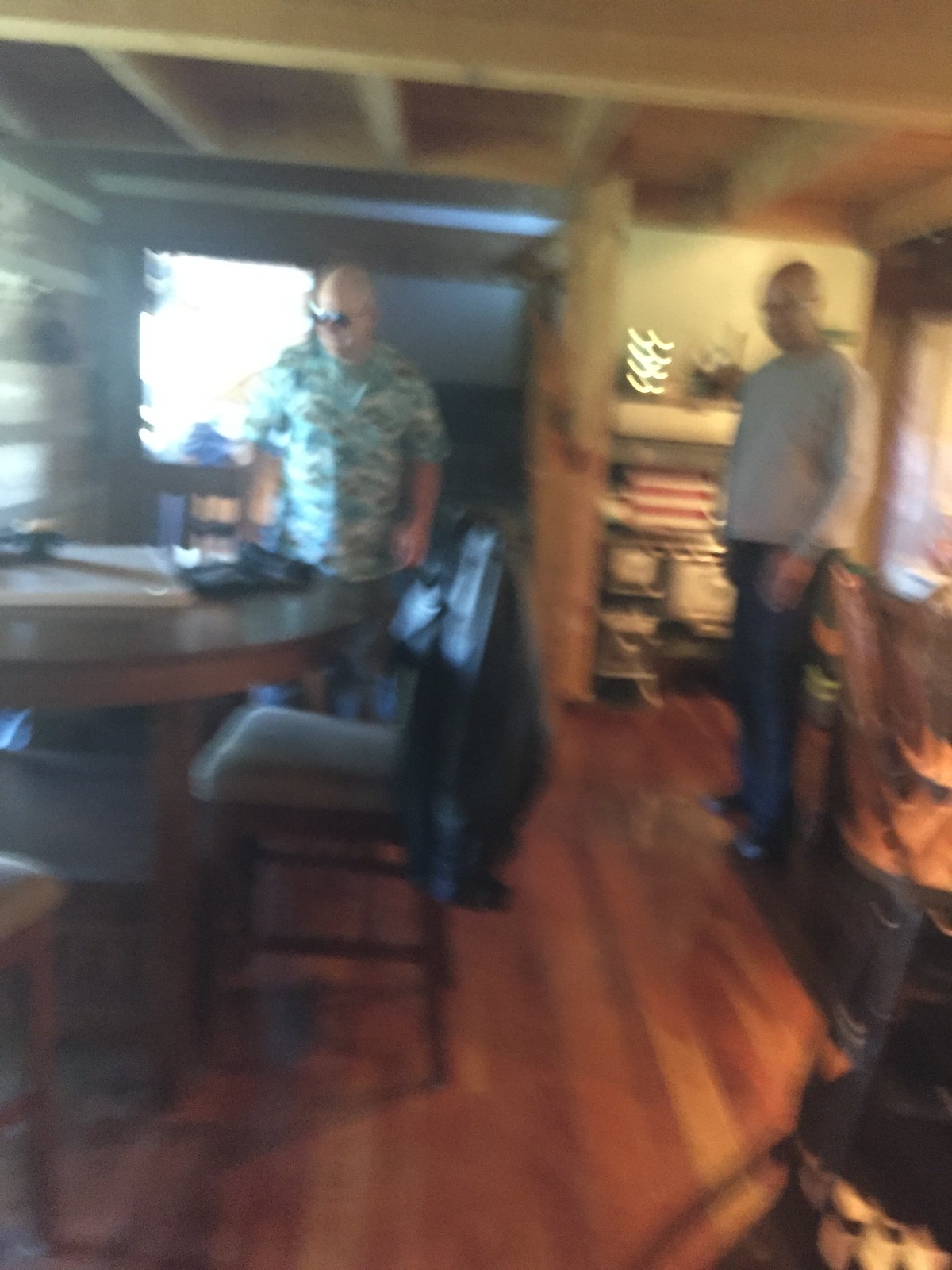The image depicts a blurry indoor scene, likely within a house or a log cabin, characterized by extensive use of wood on the floors, ceiling, and walls, contributing to its cozy, rustic feel. Central to the composition are two balding men positioned beside a round wooden table with high chairs.

The man on the left is dressed in a Hawaiian-style, short-sleeve button-up shirt and sunglasses, adding to a casual, relaxed atmosphere. Meanwhile, the man on the right sports a gray crewneck top paired with dark blue pants and black shoes, wearing regular glasses.

Amidst the somewhat cluttered background, elements such as a TV, possibly a shelf with a sculpture, and an organizer can be discerned, though the blurriness of the image makes details difficult to confirm. Additionally, the ceiling appears to have low beams, heightening the intimate, cabin-like aesthetic of the space. Both men are intently looking at something on the wooden table, which might be a tray or another object, although the exact nature of it remains indistinct.